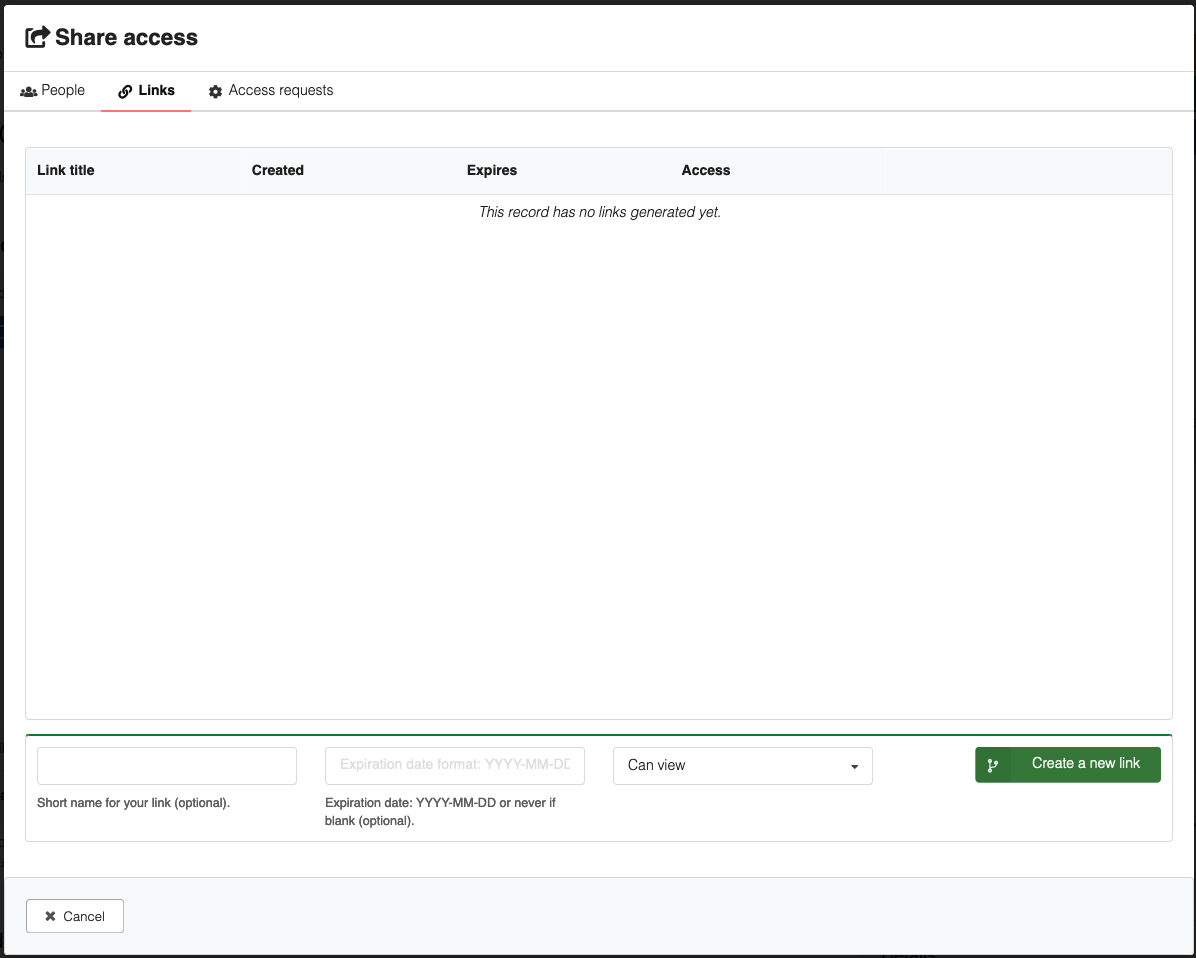A screenshot of a pop-up window titled "Share Access" appears, although the website it's associated with isn't visible. Under the "Share Access" heading are three selectable options: "People," "Links," and "Access Requests." The "Links" option has been selected. The main section of the window features an empty box with headers "Link Title," "Created," "Expires," and "Access," and within the box is the italicized text "This record has no links generated yet." Below this empty box are various input fields: a text box labeled "Short name for your link, optional" on the left, an "Expiration date or never if blank, optional" text box in the center, and a drop-down menu with "Can View" selected on the right. Positioned further to the right is a green button for creating a new link. At the bottom left of the pop-up window is a "Cancel" button.